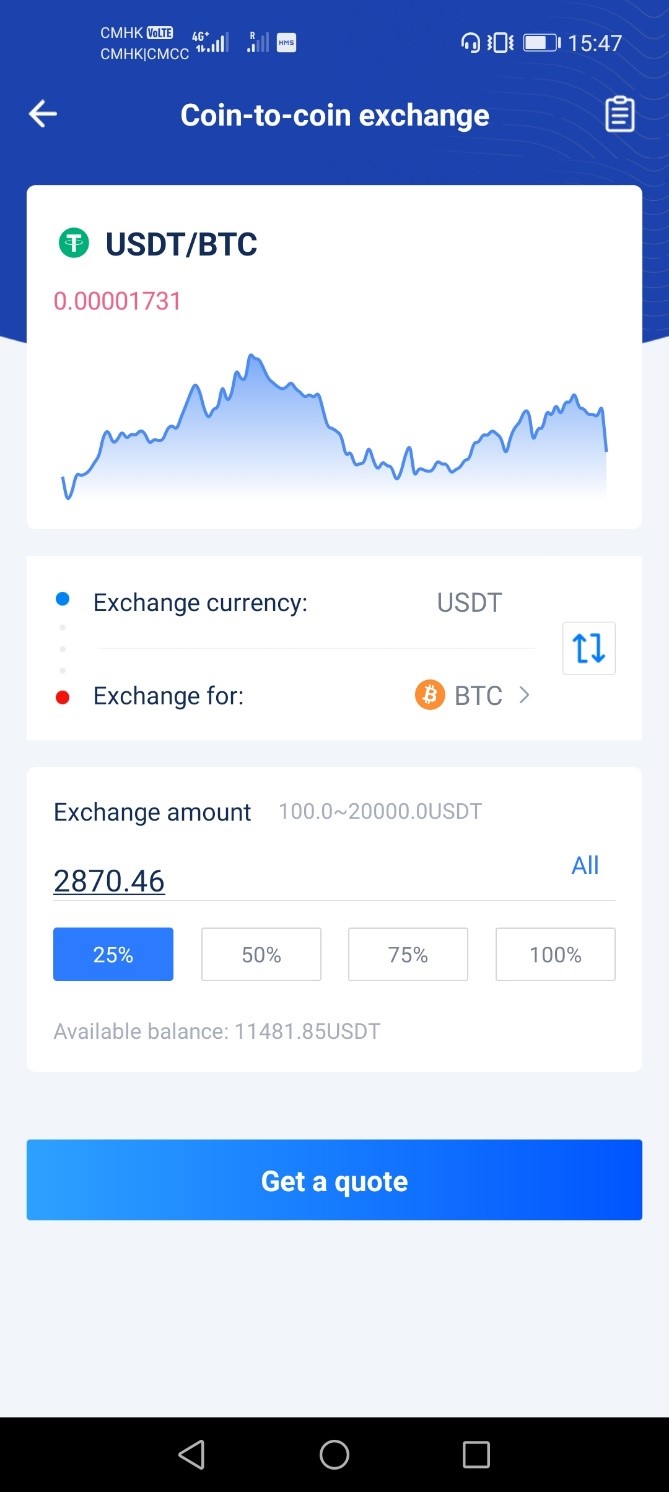The image depicts a coin exchange application interface on a smartphone screen. The user interface has a predominantly blue background.

At the very top of the screen, the title "Coin to Coin Exchange" is prominently displayed. On the top left corner, there is a large button, and on the top right corner, there is a clipboard button.

The main section below the header displays a trade pair label "USDT/BTC" on the top left, followed by a green icon with a white 'T' signifying USDT (Tether). Adjacent to this, the current price, written in red, reads "0.00001731".

Beneath the trade pair, there is a fluctuating line graph in blue, illustrating the price movement from the right side to the left side.

Towards the bottom left, there is a small blue circle labeled "Exchange Currency," beside the current currency "USDT." Adjacent to this, on the right side, there is a small red dot labeled "Exchange for BTC." The BTC icon features an orange circle with a white 'B'.

To the right side, near the middle of the screen, there is a blue shuffle button.

Below this, the section reads "Exchange amount" with a range indicated from "100" to "20,000 USDT." Further down, the number "2870.46" is displayed alongside "Oil" on the right side. Below this, a series of buttons are shown with "25%" in blue on the left, followed by "50%", "75%", and "100%" in white.

At the very bottom, it indicates "Available balance: 11481.85 USDT." Below this, there is a blue button with white text that says "Get a Quote."